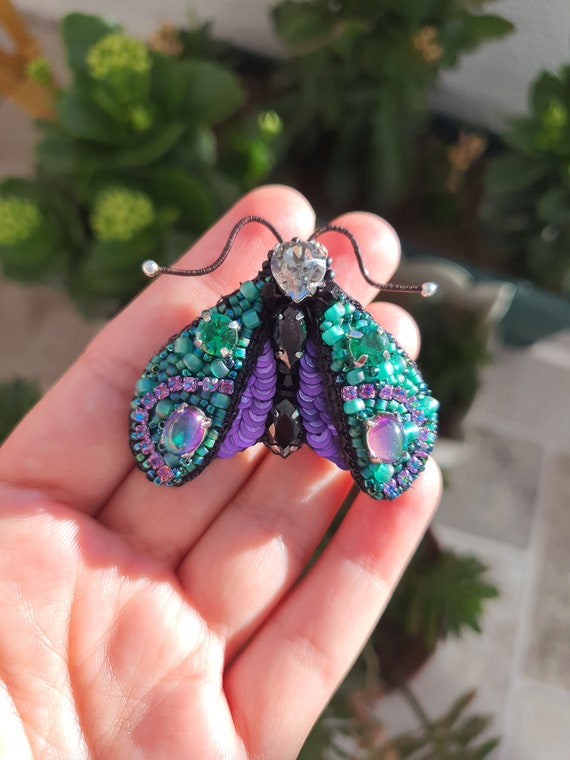The photograph features a person's left hand, angled diagonally, holding a delicate piece of jewelry that resembles a butterfly or moth-like brooch. The intricate design showcases vivid green and purple gemstone wings, with a central body composed of purple and black stones. The head of the insect is crafted from a diamond, adorned with two delicate wire antennas, each tipped with small pearl-like beads. The butterfly brooch perches near the fingertips of the hand, which is fair-skinned, with the thumb not visible in the frame. The background is a blurred outdoor scene, hinting at green plants and a stone walkway, suggesting it was taken on a sunny day as evidenced by the subtle shadows on the hand.